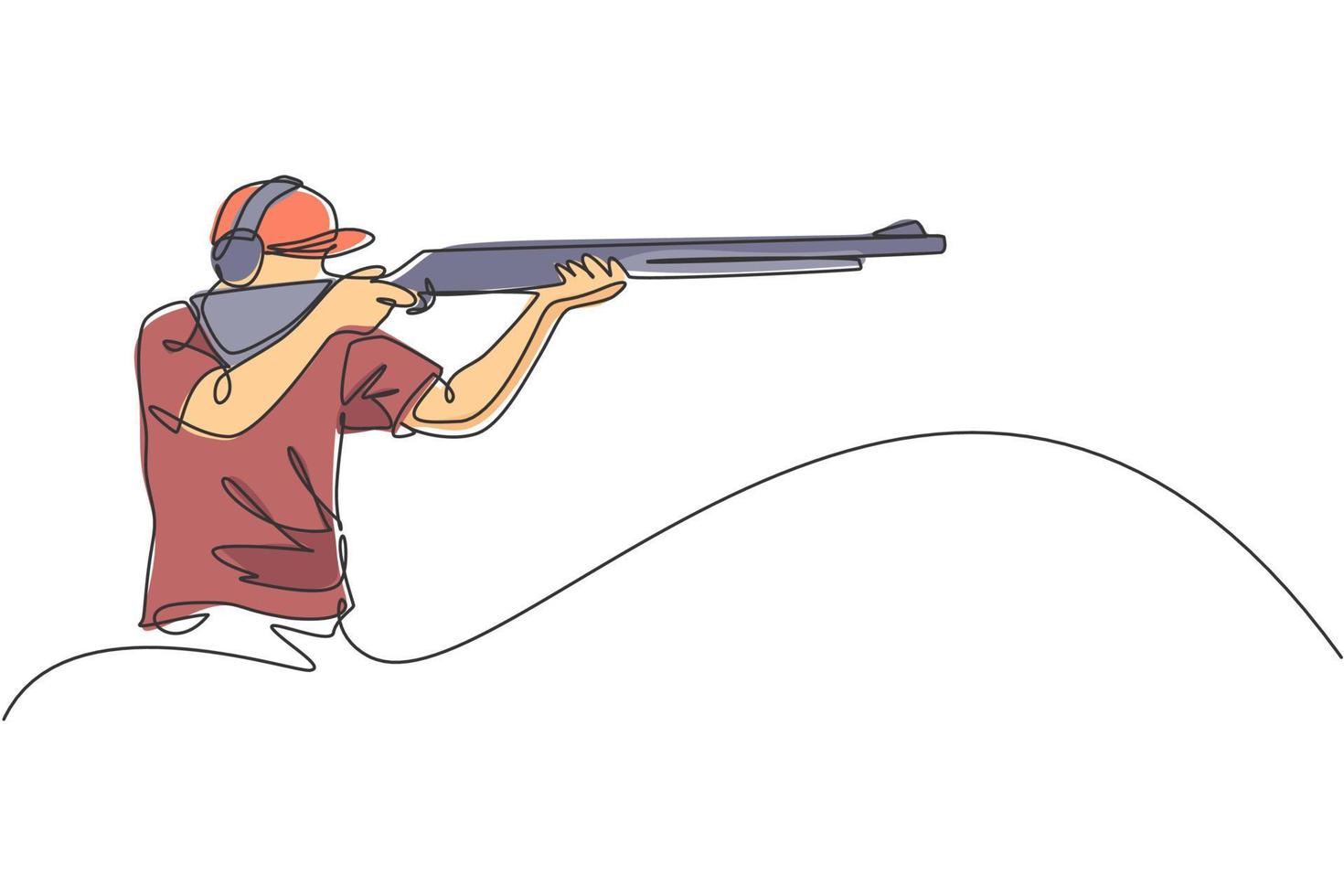This detailed sketch illustrates a young man intensely focused as he takes a shot with a long, steel-gray shotgun. Positioned on the left against a white background with a thin black outline, the man aims his gun towards the right side of the image. He is wearing a slightly wrinkled, maroon short-sleeved t-shirt and a bright orange baseball cap, along with silver protective headphones. The man, who has white skin, carefully grips the gun with one hand on the trigger and the other hand mid-barrel, peering down the sight with determination. A distinctive black wavy line, crafted in the continuous, single-line drawing style, swirls from the bottom right of his shirt, curving to the left before forming a hill shape on the right, adding an artistic touch to this captivating minimalist sketch.